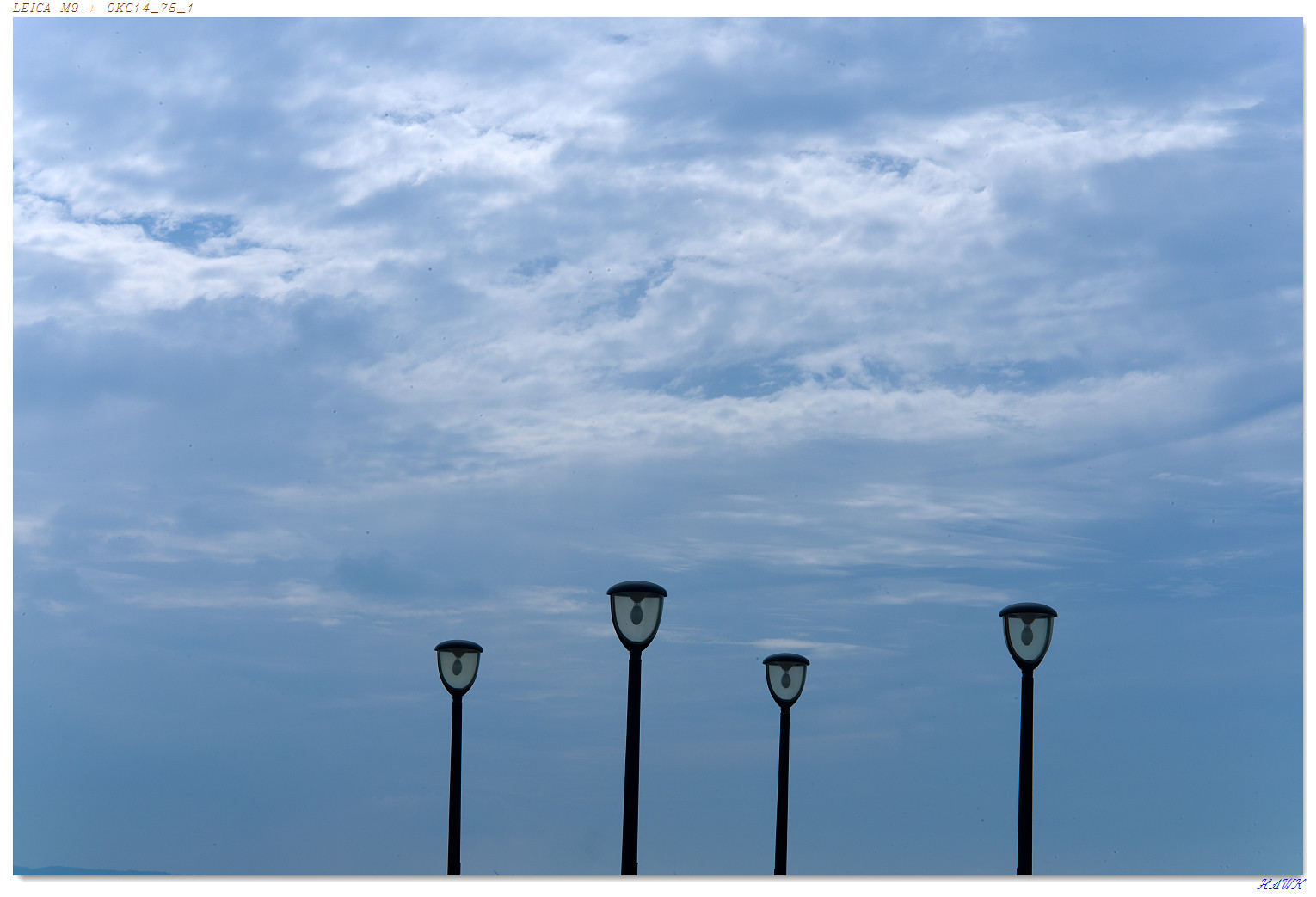The image captures a tranquil scene dominated by a blue sky dotted with white clouds, giving a serene and minimalist feel. In the foreground, four evenly spaced black lampposts stand tall with only their top thirds visible. Each lamppost features a thin black pole supporting a glass housing bordered in black, topped with small rounded black domes. The transparent glass distinctly reveals the light bulbs inside, forming an hourglass-like silhouette. The light bulbs are currently off, emphasizing the peacefulness of the sky above. There are two watermarks present; one in the bottom right corner reading "K-A-W-X Cox" and another in the top left corner that appears to say "L-E-I-C-A-M-9-O-K-C-J-1-4_7_5_1." The overall composition focuses on the vastness and tranquility of the sky, merging the earthly structures seamlessly with the ethereal backdrop.